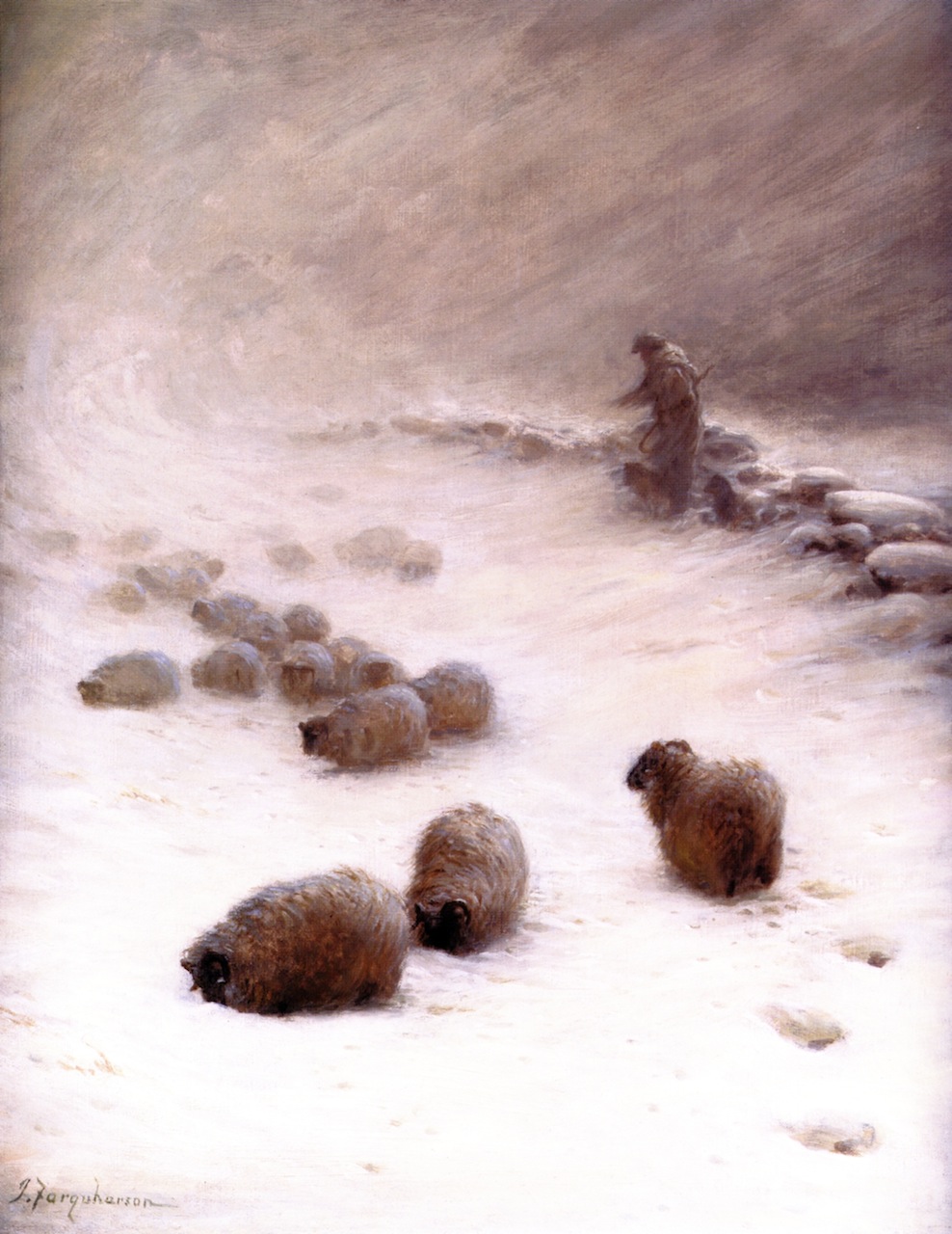This painting vividly depicts a snow-laden landscape where a shepherd is tending to a large flock of sheep during a blizzard. The scene is almost monochrome, dominated by shades of white and brown, with intricate brush strokes that convey the violent, swirling wind of the snowstorm. The shepherd, dressed in a brown jacket and pants, stands at a rocky outcropping, a shepherd's hook in hand, looking left and seemingly engaged with the environment. He is surrounded by his woolly, fluffy sheep, many of which are knee-deep in snow, leaving visible footprints behind. The sheep, mostly brown in color, appear more white and possibly buried in snow on the top right of the image, blending with what might be snow-covered rocks. The entire scene is framed by a rock fence and a hill or cliff in the background. The painting captures the harshness of the blizzard and the resilience of both the shepherd and his flock. There’s a faint signature in the lower left-hand corner, adding a touch of mystery to the artist's identity.